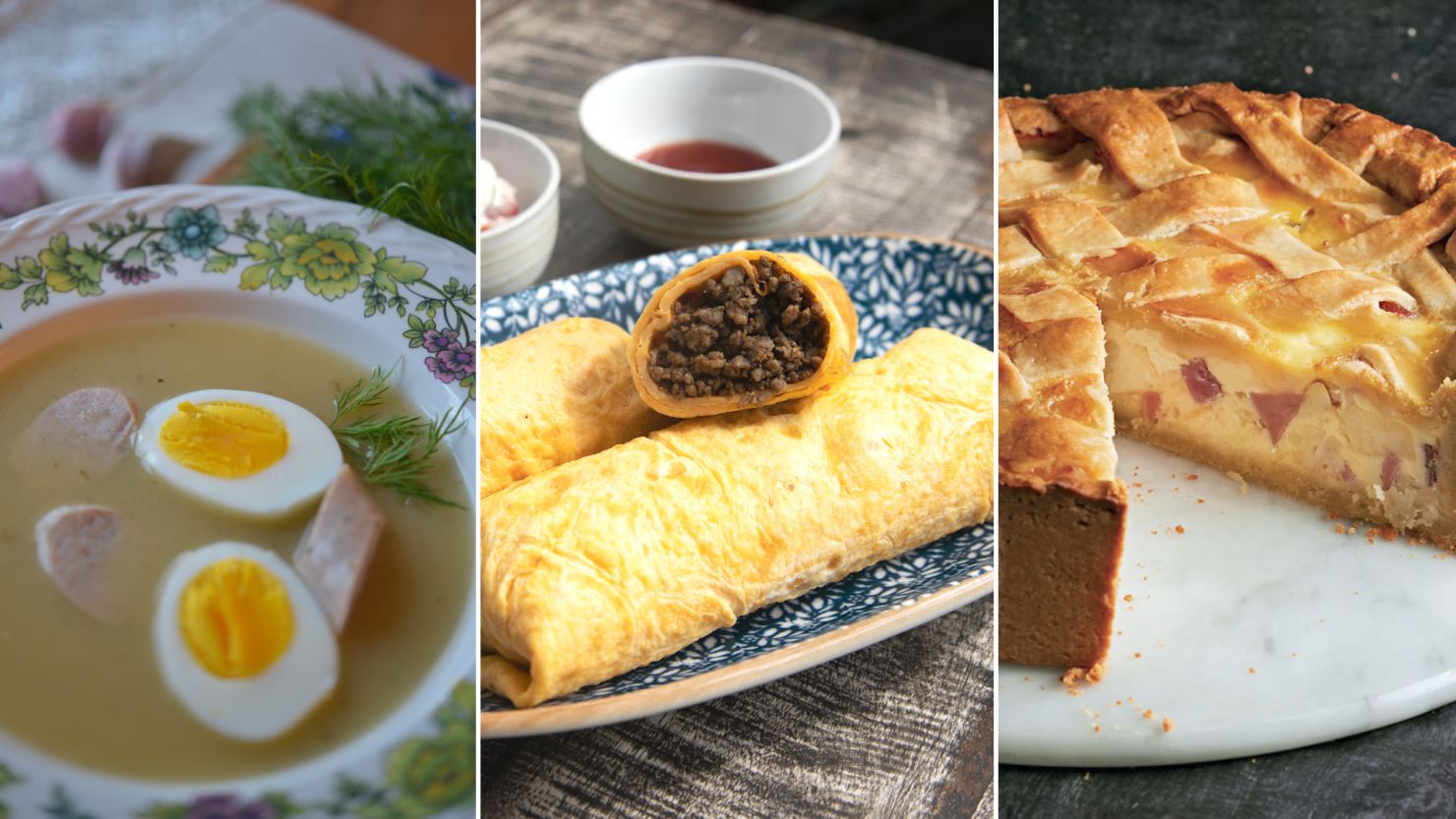The image showcases three distinct food dishes artfully arranged on plates, presented in a horizontal layout. On the left, a floral-patterned bowl encases a golden chicken broth, featuring a halved hard-boiled egg, chunks of savory sausage, and a sprig of green herb, likely dill. The middle dish consists of a trio of burritos or deep-fried tortillas filled with ground beef. One burrito is sliced open to reveal its rich brown meat filling, all arranged on a blue and white platter. Behind them, two small bowls hold a deep red dipping sauce and possibly sour cream. The final dish on the right is a beautifully baked quiche with a golden lattice crust, resembling a traditional pie. The filling comprises eggs, likely potatoes, and bits of meat or tomato, all served on a marble plate.